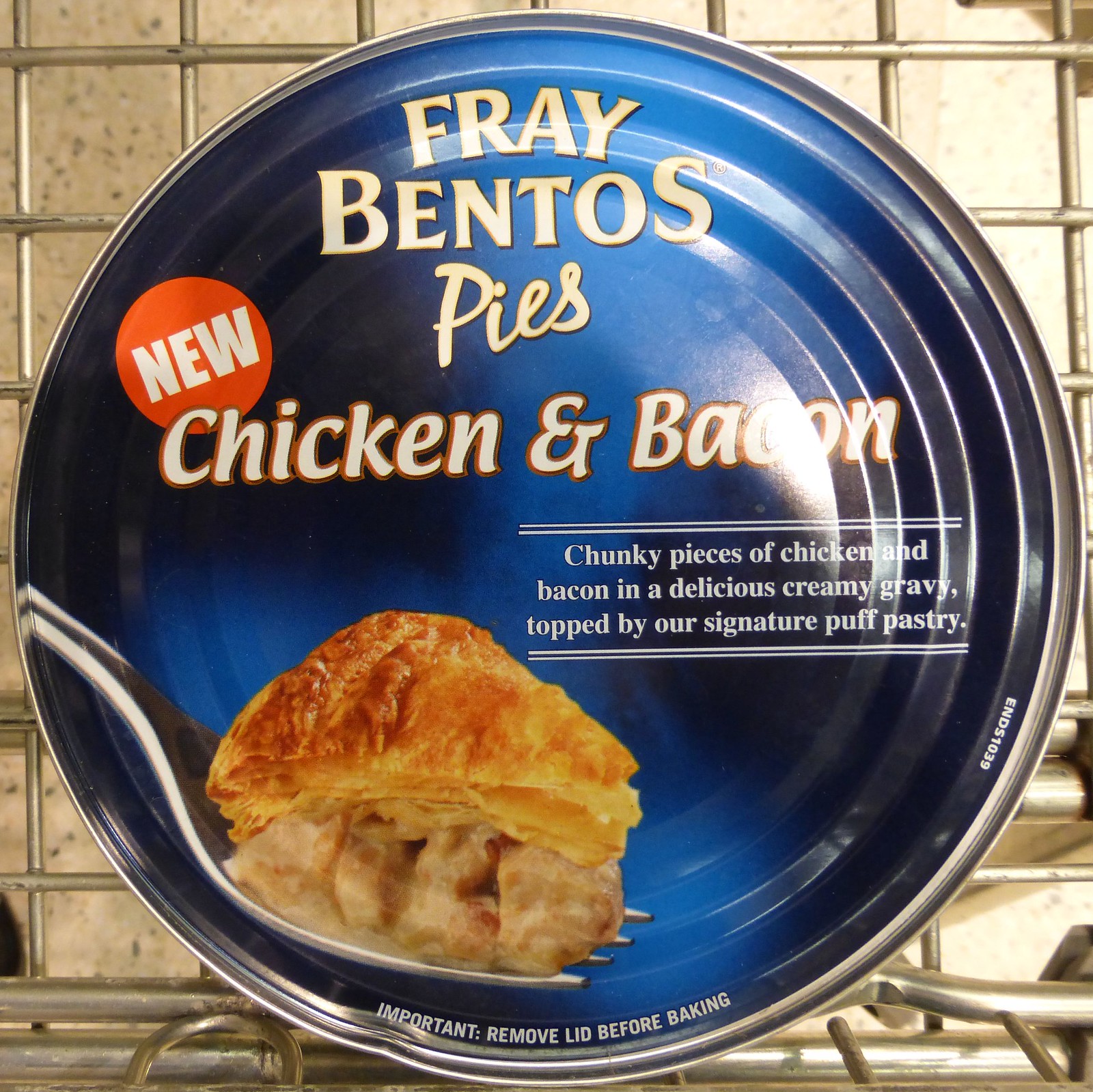This indoor photograph centers on a prominently displayed can of Frey Bento’s Pies, specifically the Chicken and Bacon variety. The can, topped with a mix of blue and black colors, features a detailed label and a vibrant banner. The text reads: "Frey Bento's Pies Chicken and Bacon. Chunky pieces of chicken and bacon in a delicious creamy gravy topped by our signature puff pastry." A tempting image shows a piece of the pie on a fork, emphasizing the creamy gravy and chunky meat. To the left of the can is a striking red circle with the word "new" in white font, indicating a new product variation. Below the can, there appears to be a metal grate or cooling rack, possibly part of a grocery cart. The can itself, though slightly dented near the bottom left side, looks shiny and likely unopened, adding to the pristine display of the product. A small white text at the bottom reminds consumers to "Important: Remove lid before baking."